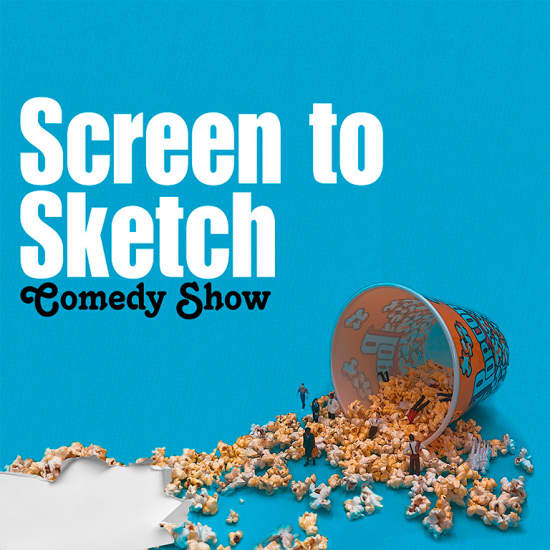This vibrant advertisement poster features a playful design promoting a comedy show titled "Screen to Sketch." Set against a bright baby blue background, the large, bold white text announcing the show's title dominates the top section of the poster. Below it, in smaller black text, is the subtitle "Comedy Show." The central visual element is an oversized, tilted orange popcorn bucket with white writing, dramatically spilling popcorn across the foreground. Among the scattered popcorn, miniature action figures are whimsically posed—some standing, walking through the popcorn, while others lie buried or half-tumbled out of the bucket, creating a dynamic scene. The bottom left corner of the poster features a jagged tear effect, revealing a white background beneath the blue, adding an extra layer of visual interest. This creative composition effectively captures the lively and humorous spirit of the event being advertised.